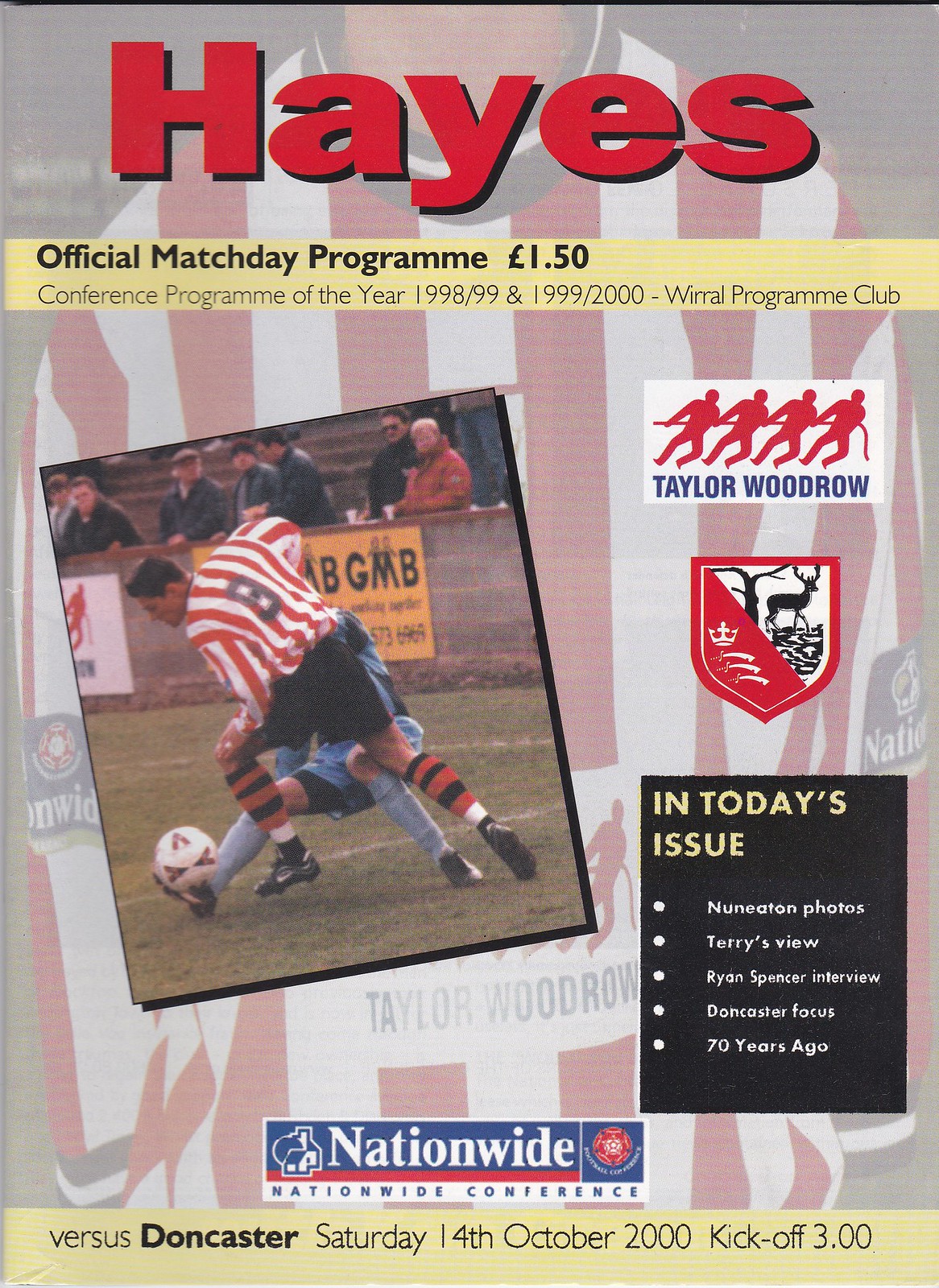The image is a detailed cover of a soccer program. At the top, prominent red text with a black drop shadow spells out "HAYES" (H-A-Y-E-S). Beneath this, a yellow banner with black text announces, "Official Match Day Program, £1.50" (wording varies slightly in different quotes), followed by "Conference Program of the Year 1998/99 and 1999/2000" and "World Program Club." 

Toward the center-left of the cover, there is a picture of a soccer player in action, wearing a red and white striped shirt with "Taylor Woodrow" displayed on the front, black shorts, and red and black striped socks. The player is positioned to kick the ball, while another player, dressed in a blue and black uniform, appears to be falling at his feet. 

On the right side of the cover, there's text that reads "In Today's Issue," which previews the magazine's content. Below this, a logo featuring four red figures pulling on a rope is visible, and nearby is a red shield logo with a white corner. The background shows spectators watching the game. The entire composition is lively, depicting the dynamic atmosphere of a soccer match.